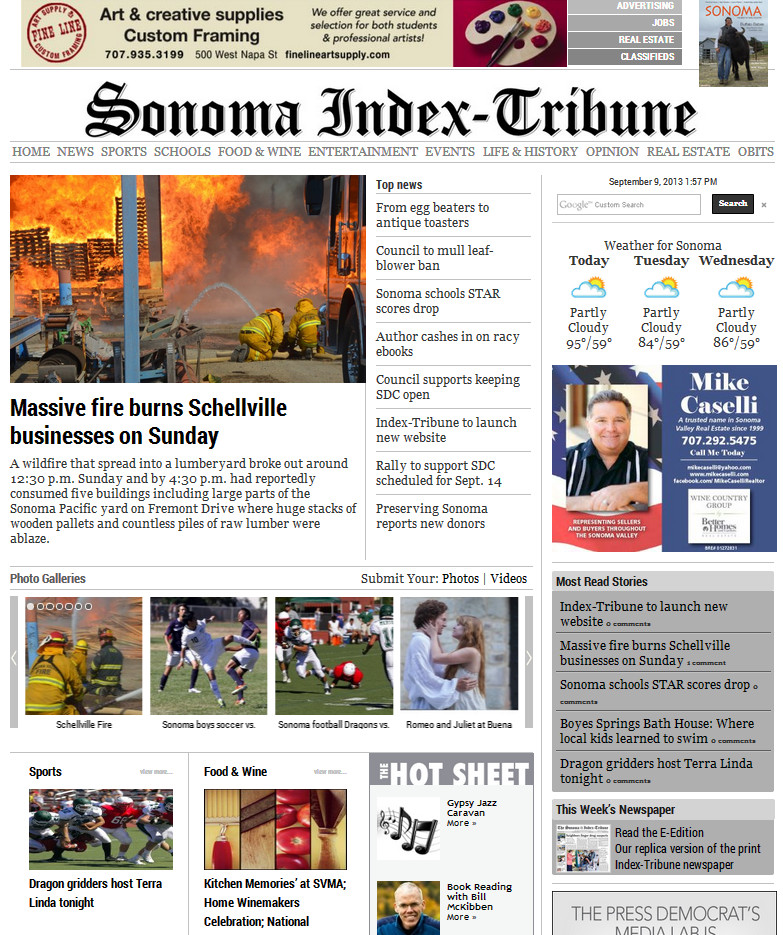Front page of the Sonoma Index Tribune:

At the very top, a banner for an art supply store reads: "Art and Creative Supplies Custom Framing. We offer great service and selection for both students and professional artists. 707-935-3199, 500 West Napa Street, finelineartsupply.com." The banner is accompanied by a photograph of a white palette filled with numerous colors of paint and a paintbrush resting on the side, set against a red surface. 

Adjacent to the banner, the newspaper offers links to sections such as Advertising, Jobs, Real Estate, and Classifieds.

The newspaper's name, "Sonoma Index Tribune," is presented in an Old English font, with navigation options like Home, News, Sports, Schools, Food and Wine, Entertainment, Events, Life and History, Opinion, Real Estate, and Obits listed below it.

Dominating the front page is a dramatic photograph of a raging fire being fought by firemen. The accompanying headline reads: "Massive fire burned Shellville businesses on Sunday." The article briefly details that a wildfire broke out around 12:30 p.m. at a lumberyard and by 4:30 p.m. had consumed five buildings, including large parts of the Sonoma Pacific Yard on Fremont Drive.

To the right of the fire headline, a section labeled "Top News" features several stories, including:
- From egg beaters to antique toasters
- Council to mull leaf blower ban
- Sonoma School star scores drop
- Author cashes in on racy e-books
- Council supports keeping SDC open
- Index Tribune to launch new website
- Rally to support SDC scheduled for September 14th
- Preserving Sonoma reports new donors

Additional sections include "Photo Galleries" with prompts for readers to submit their photos and videos of events like the Shellville Fire, Sonoma Boys Soccer, Sonoma Football Dragons, and a performance of "Romeo and Juliet at Buena."

In the "Sports" section, the headline reads: "Dragon Gritters host Tara Linda Tonight."

In "Food and Wine," there's mention of events like "Kitchen Memories at SVMA" and the "Home Winemakers Celebration."

"The Hot Sheet" lists upcoming events such as:
- Gypsy Jazz Caravan
- Book reading with Bill McKibben

On the right-hand side of the page:
- The date and time: September 9th, 2013, 1:57 p.m.
- A Google Custom Search field
- Local weather forecast for Sonoma: partly cloudy with high temperatures of 95°F/59°F today, 84°F/59°F on Tuesday, and 86°F/59°F on Wednesday.

A photograph of a middle-aged man smiling with his hands folded in front of him is set against the backdrop of an American flag. The caption reads: "Mike Caselli, a trusted name in Sonoma Valley real estate since 1999, representing sellers and buyers throughout the Sonoma Valley. 707-292-5475, call me today."

"Most Read Stories" includes:
- Index Tribune to launch new website
- Massive Fire burns Shellville businesses on Sunday
- Sonoma Schools star scores drop
- Boys Springs Bath House where local kids learn to swim
- Dragon Gritters host Tara Linda Tonight

Finally, there's an invitation to read "This week's newspaper" or the e-edition, which is the replica version of the printed Sonoma Index Tribune newspaper.